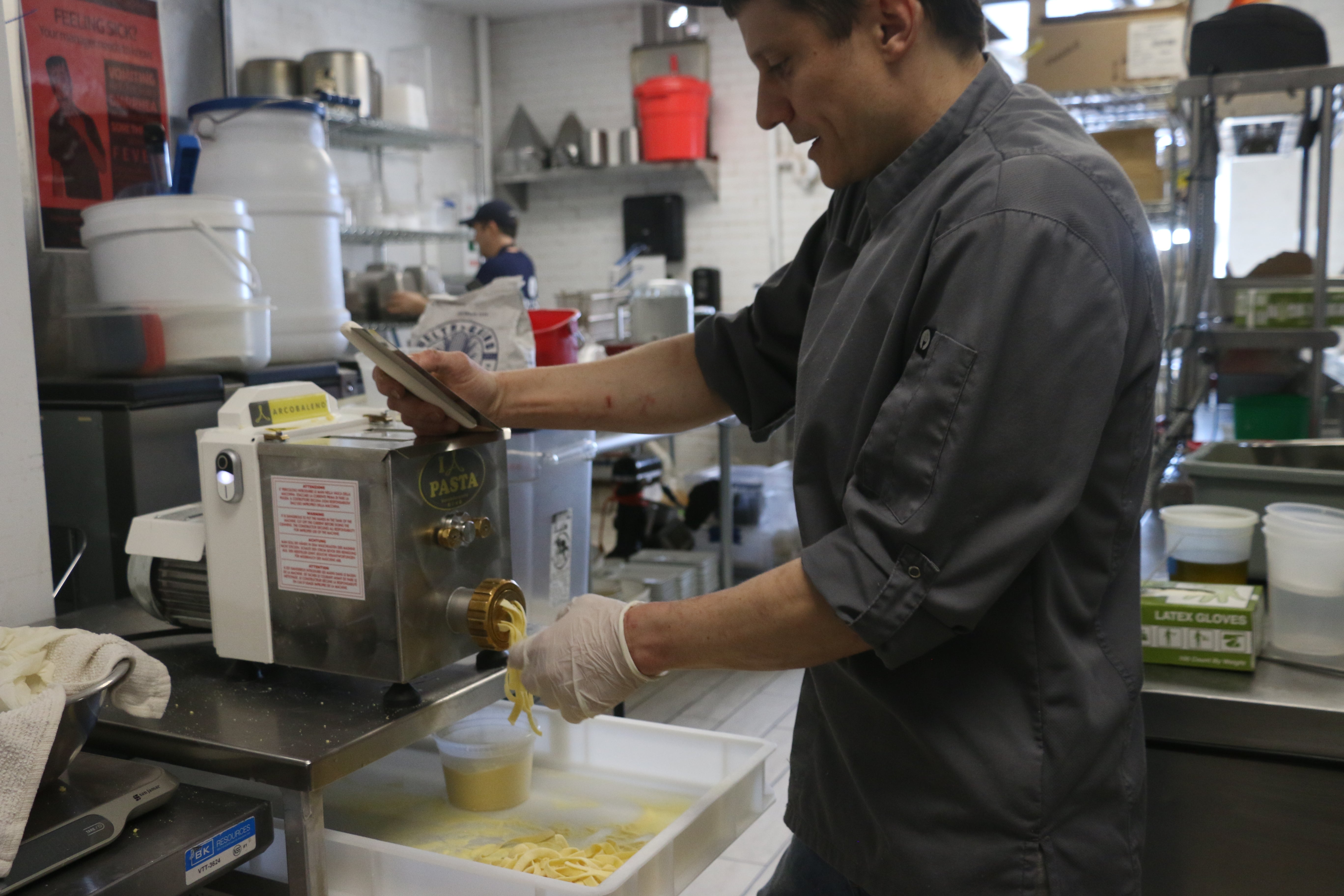In a bustling commercial kitchen, a chef in a gray outfit stands at the forefront, meticulously operating a pasta maker. Wearing white gloves, he expertly catches the freshly extruded pasta and places it into a white tray below the machine. He momentarily glances at his phone held in one hand while managing the pasta with the other. The kitchen, characterized by its white walls and floor, is filled with various culinary equipment and storage solutions. Shelves are stocked with pots, pans, and white plastic buckets, while stainless steel surfaces glisten under the bright lights. Directly behind the chef, another worker is partially visible in the distance, wearing a baseball hat and a dark t-shirt, possibly washing dishes. A large window at the far wall allows sunlight to stream into the room, adding a touch of natural light to this professional culinary space.